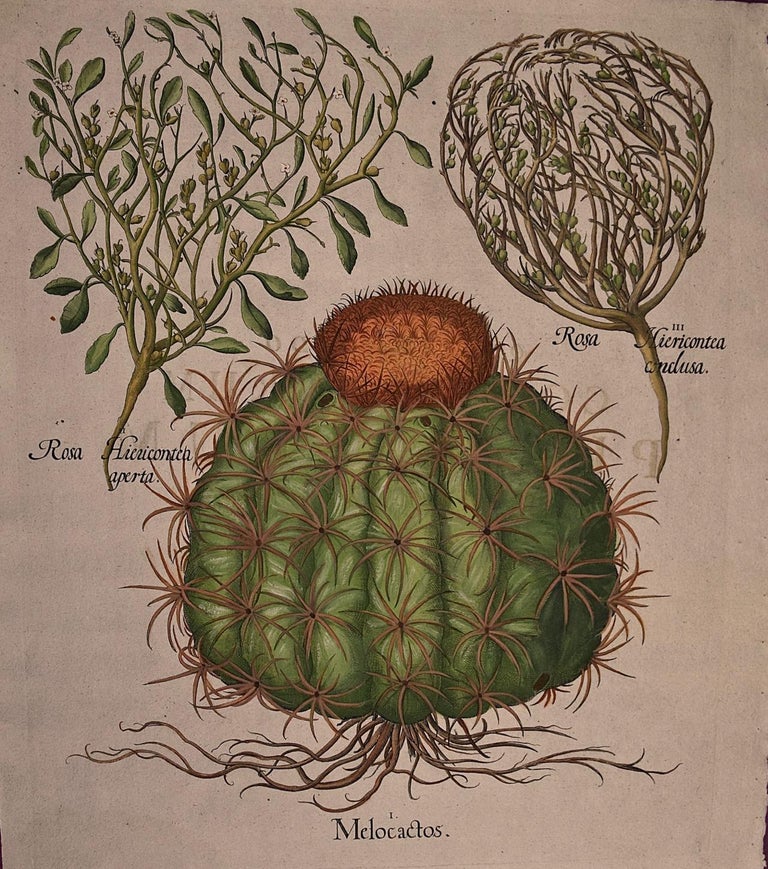This exquisitely detailed portrait-format illustration, presented in color, features a botanical study with antique aesthetics, reminiscent of a vintage manuscript. The focal point is a "Mellow Cactus," labeled as such at the bottom of the image. The cactus itself is green, round, and adorned with small spikes. Topping it is an intriguing orange ball, possibly a spiky fruit or a miniature cactus. The background is light pink, enhancing its antique and Victorian-style appearance, including the Latin labels which add to its historical charm.

To the top right and top left of the main cactus, there are two supplementary illustrations of plant species: Rosa hiracanta aperta and Rosa miracantia inclusa. These illustrations feature stems with green leaves and branches which might be connected or related to the main cactus species. The drawing technique appears to be colored pencil, adding richness and texture to the illustration. This whole setup is presumably a photograph of a page from a botanical book, capturing the enchanting blend of science and artistry in plant representation.